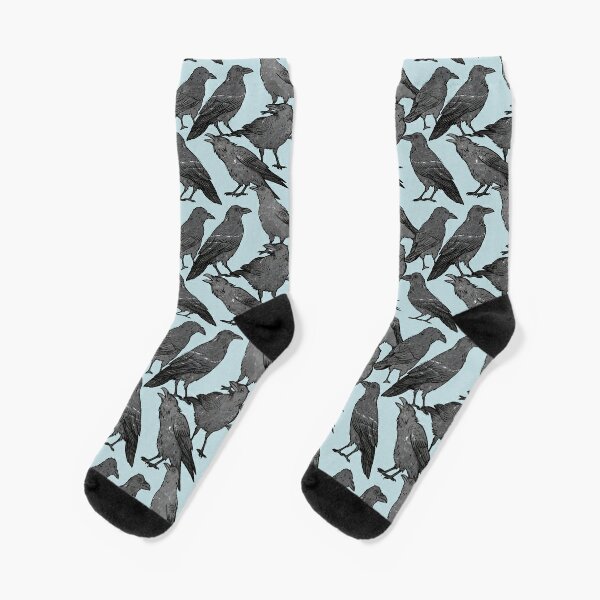The image depicts a pair of light blue, calf-length socks laid out flat on a solid white background. The socks are adorned with numerous black crows scattered throughout the entire surface. Each crow is rendered in varying poses—some are cawing, some staring, and others just sitting still, giving a dynamic feel to the design. The heel and toe portions of the socks are solid black, matching the color of the crows. The background of the image casts a faint drop shadow, enhancing the visibility and contrast of the socks against the white surface.